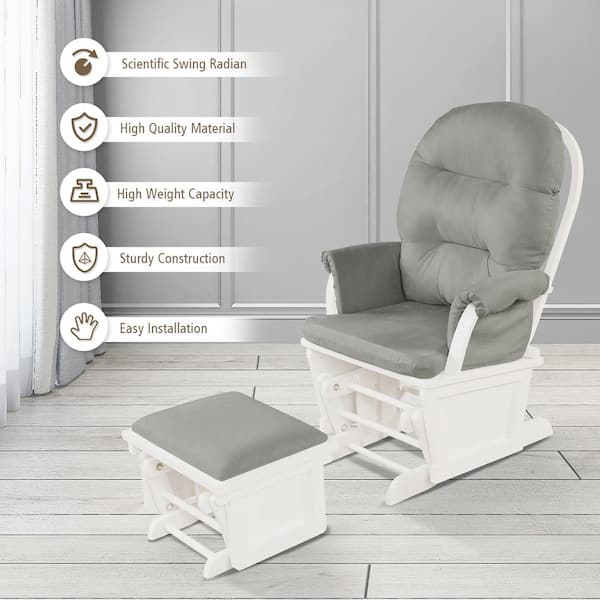In this black and white photograph, the focal point is a glider rocker and an ottoman positioned in the middle of a room. The glider rocker has a white wooden base with medium gray cushioning, and the matching ottoman also features a white base and a medium gray cushion. The floor is styled with gray wooden pieces, matching the gray hue of the walls. To the left side of the image, partially overlaid on drapes, are five icons accompanied by text, presumably added in post-processing. The text details the product features, listing "scientific swing radian," "high quality material," "high weight capacity," "sturdy construction," and "easy installation." Both the rocker and the footstool are set at an angle, enhancing the view of their design and features.